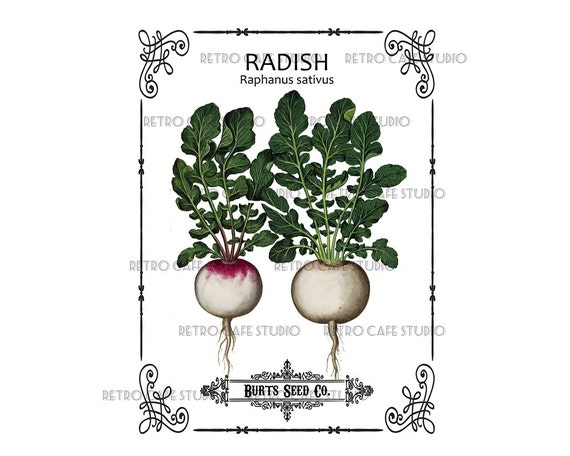The image is a vertically-oriented, old-fashioned seed packet illustration featuring two radishes, labeled "Radish Raphanus sativus" at the top. The radishes are centered, with one predominantly white and the other with a red-tinted top. Both have detailed green leaves sprouting and visible roots. Surrounding the radishes is a thin, black ornate border decorated with curlicues and L-shaped designs in the corners. At the bottom, in elegant cursive, it says "Burt's Seed Co," encased in an intricate black filigree. The background is white, and there are multiple faint imprints of "Retro Cafe Studio" scattered throughout the image, adding a textured, vintage feel.